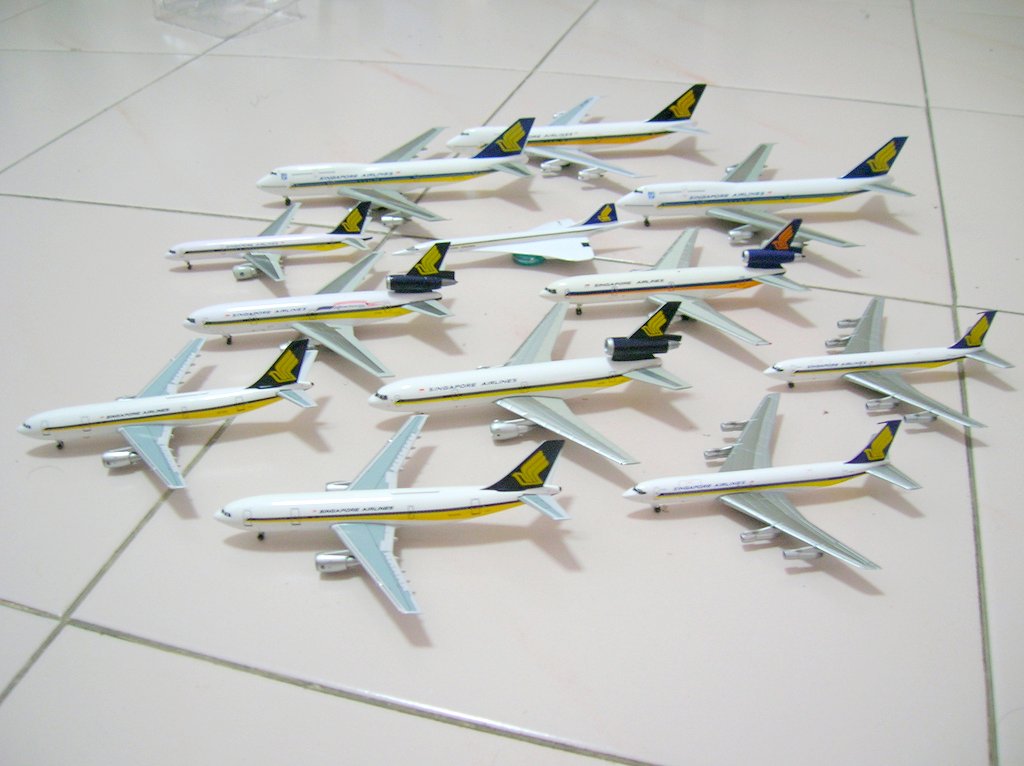This image showcases a collection of twelve toy airplanes, predominantly modeled after Singapore Airlines aircraft. The planes are arranged on a white tiled floor with a grayish grout, possibly in a home or display setting. They are aligned parallel to each other, all pointing to the left. Each plane is characterized by a white body with a single blue stripe running along the middle and a yellow underside. The tail features the distinctive Singapore Airlines yellow flight symbol, although one plane has a red flight symbol and a blue turbo jet component. Despite slight variations, such as one plane having a flatter shape, they collectively present a cohesive and orderly display.